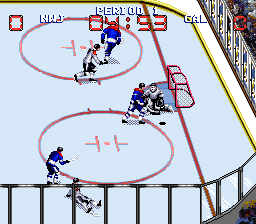This small, square illustration captures a nostalgic moment from an older style video game, reminiscent of the classic Game Boy era. The scene depicts a hockey game, characterized by its pixelated graphics and simple, vivid color palette featuring primarily reds, whites, blues, yellows, and grays. On a rink of ice, six players are engaged in the game, divided into a blue team and a white team. Dominating the rink are two large red circles and a red line leading to a goal post, setting the stage for the on-ice action. At the upper center of the image, a timer displays "0493," and red text on either side shows a score of "0-0." Above this, the label "Period 1" is prominently placed, indicating the game's progress. The overall illustration is a charming throwback to retro video game aesthetics, complete with basic yet evocative designs and colors.